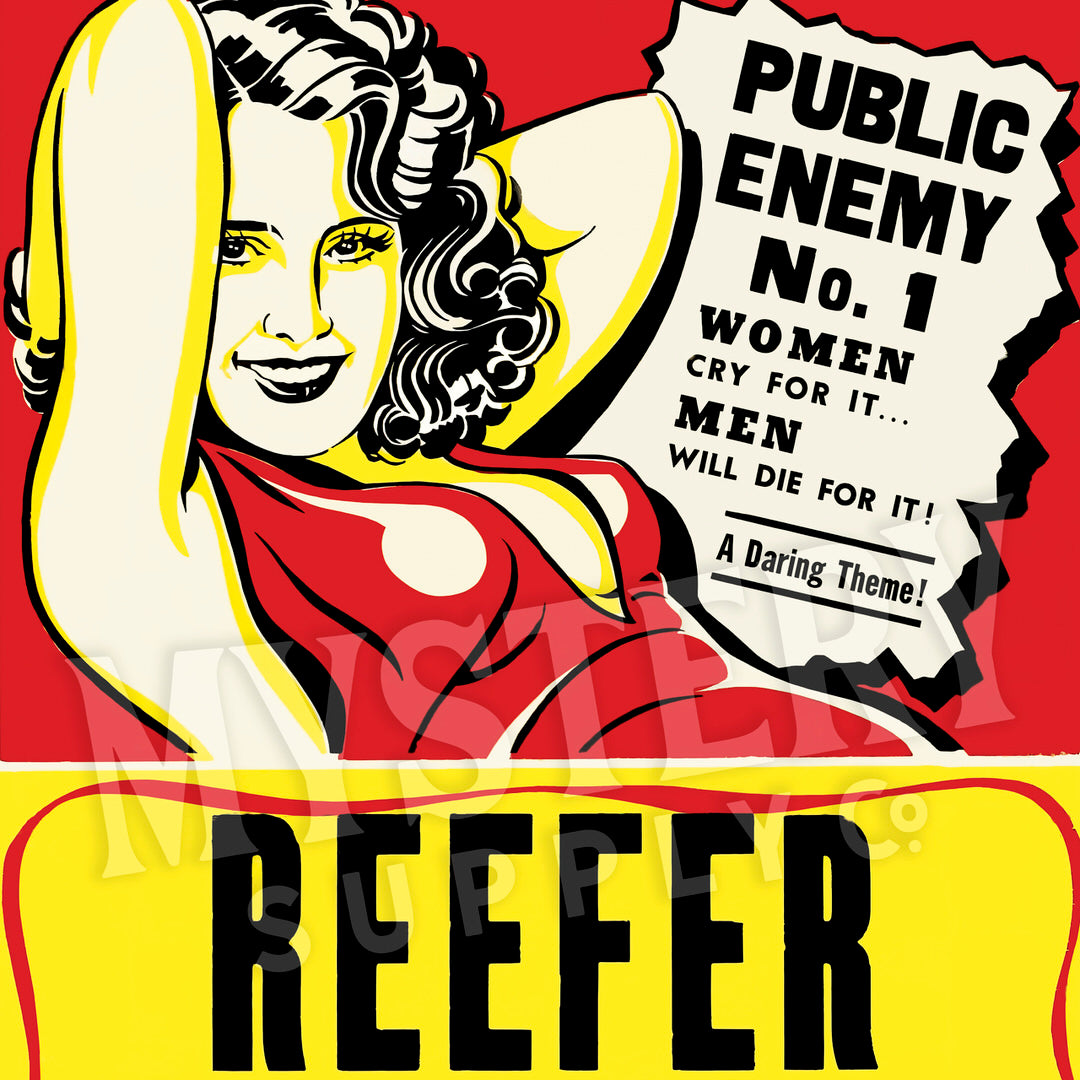The image presents a vibrant and striking poster reminiscent of vintage magazine or comic book covers. Dominating the left side is a detailed cartoon-style drawing of a beautiful young woman with shoulder-length curly black hair, outlined in yellow and with white skin. She is smiling and looking directly at the viewer, her red lipstick accentuating her expressive face. Dressed in a sleeveless, deep-neck red dress that reveals her cleavage, she has her hands raised, exposing her armpits.

Adjacent to her, on the right side, is a white box designed to resemble a torn piece of paper. Written in bold black letters, the text within the box reads: "PUBLIC ENEMY NUMBER ONE, WOMEN CRY FOR IT, MEN DIE FOR IT, A DARING THEME." Below this, there is a yellow horizontal strip, bordered with a red ribbon-like design. The strip features large, capitalized black text that reads: "REFER." The entire background of the image is a vivid red color, contributing to the overall pop-art aesthetic. Additionally, the image includes a subtle transparent watermark that reads "Mystery Supply Company."